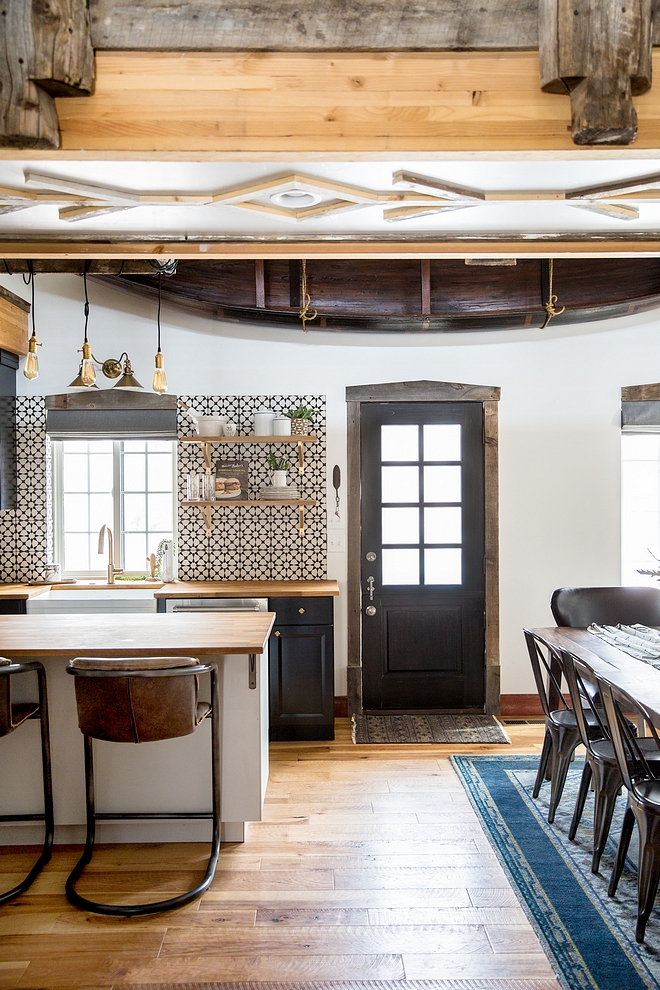This image showcases the picturesque interior of a cozy cabin-style home. On the left, the kitchen area features a sophisticated tile backsplash in dark blue and white hues. The kitchen boasts two open shelves adorned with various containers and bowls. Above the sink, three elegant Edison lights dangle from the ceiling, illuminating the space. The bronze kitchen sink, equipped with a swan neck faucet, complements the butcher block countertops and contrasting black cabinets. A peninsula with a brown wood top and a white base provides additional workspace. Positioned against the peninsula are two modern leather chairs with black metal supports, designed to swing out behind them. 

The wooden floors extend into a dining area to the right, where a blue area rug anchors the space. A rustic wood plank dining table sits atop the rug, surrounded by three black café-style chairs and a larger chair at the head of the table. Through a partially visible window, natural light filters into the room.

In the background, a striking black door with eight small square windows on its upper half stands out. Suspended from the ceiling is an intriguing canoe, adding a touch of character to the room. The ceiling itself features exposed wood beams, along with a section of light wood edges and recessed lighting. Thin wooden boards arranged in a pattern add an additional element of warmth and texture to the ceiling, completing this charming and meticulously designed cabin interior.